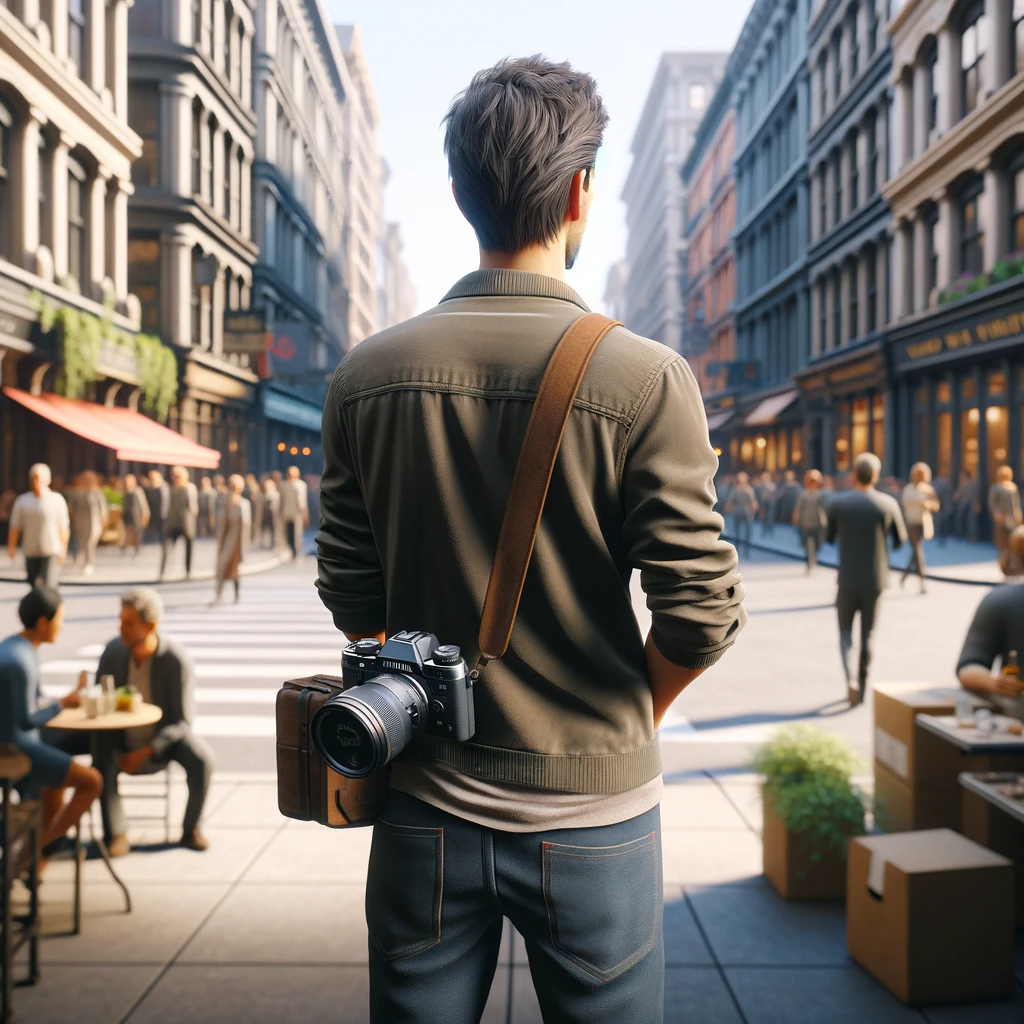The image, possibly AI-generated or graphically designed, depicts a young man with short black hair and a brown jacket over a white t-shirt. He is wearing blue jeans featuring two back pockets. Standing with his back to the viewer, he occupies the center of the frame. A vintage 35-millimeter camera hangs from a brown strap over his shoulder, resting against his hip, and he carries a small case on his left side. He faces a street scene with a pleasing, vintage color palette dominated by greens and blues. On either side, the sidewalks are busy with people walking and others seated at tables enjoying meals. The street is lined with shops and buildings ranging from four to ten stories, lending a sense of architectural sameness that's aesthetically pleasing overall. The background appears slightly blurred, emphasizing the young man as the focal point of the image.